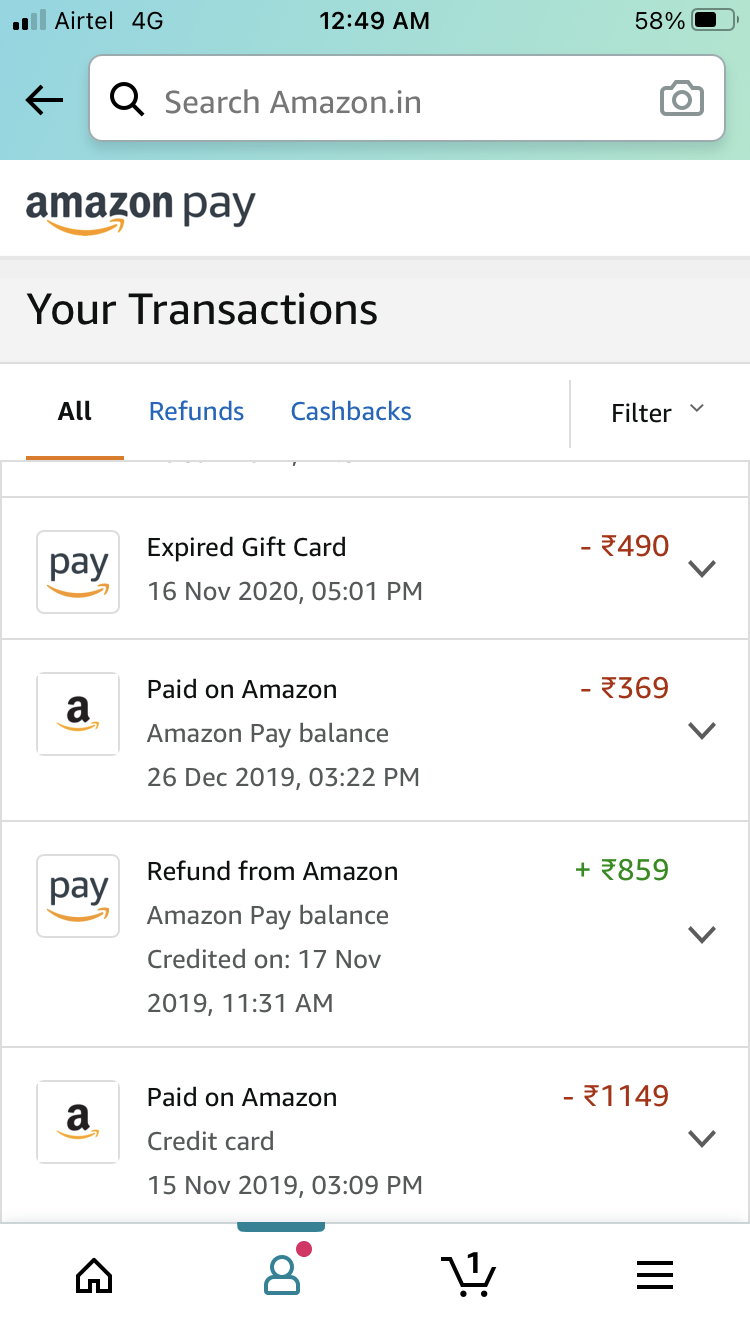In this image showcasing the Amazon app, the top section features a distinctive blue bar with a black back arrow on the left. Centrally positioned at the top is a search box. Below this, the Amazon logo is prominently displayed, accompanied by the word "Pay" next to it. Directly beneath, there is a gray box labeled "Transactions," followed by three tabs: "All," "Refunds," and "Cashbacks," with the "All" tab currently selected. To the right of these tabs, a filter drop-down menu allows users to refine their search within the transactions. Below this section, several transactions are listed: a payment involving an expired gift card for 490 rupees, another payment on Amazon for 369 rupees, a refund from Amazon amounting to 859 rupees, and yet another payment on Amazon for 1149 rupees.